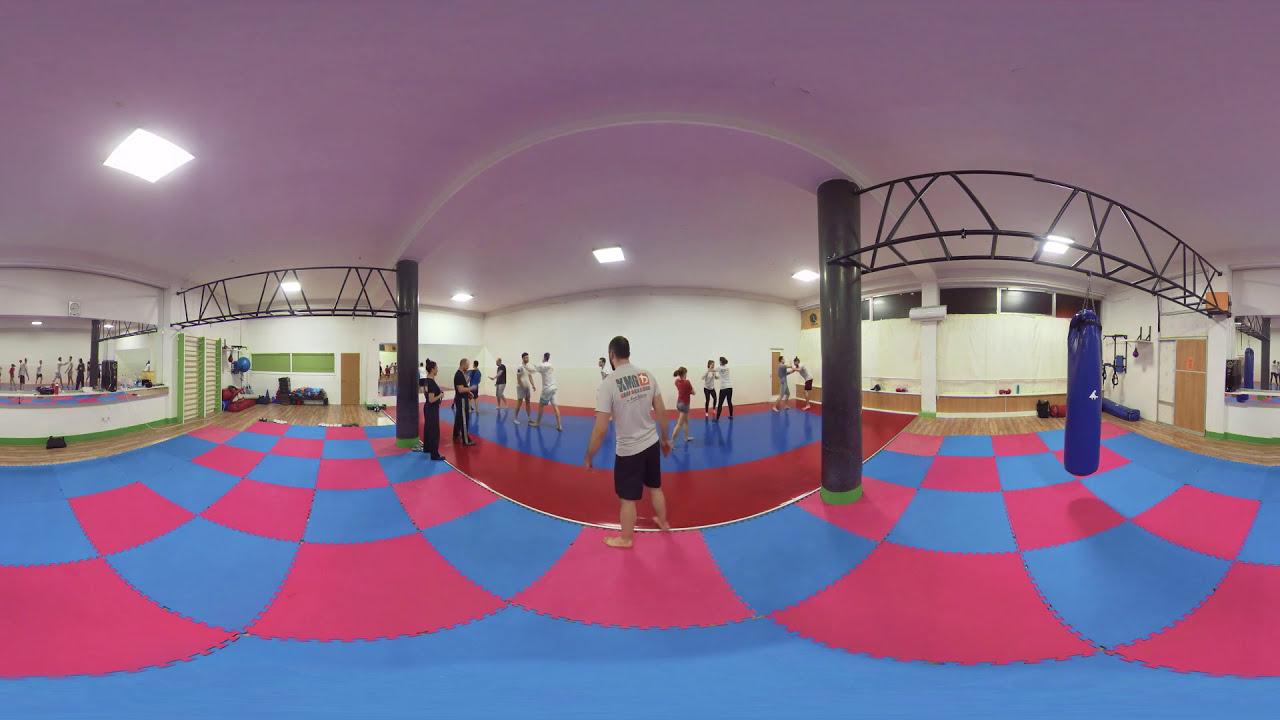The image captures a vibrant and expansive panorama of an indoor martial arts gym. The floor is a distinctive checkerboard pattern in blue and pink, made of interconnected rubber mats reminiscent of puzzle pieces. This striking pattern gives way to a smoother, tiled flooring towards the back of the gym. 

Throughout the gym, there are several pairs of adults, barefoot and casually dressed, engaged in sparring exercises. They appear to be practicing various self-defense and martial arts techniques, such as punching, holding, and wrestling. In the middle of the scene stands an instructor with black hair and a beard, identifiable as a coach by his shirt emblazoned with the initials "KMG." His back is turned to the camera as he oversees the training session.

The gym is equipped with various martial arts apparatus, including hanging punching bags attached to wire frames and pillars. A dark blue punching bag is notably positioned on the right side of the image. The environment is mirrored, enhancing visibility and allowing participants to observe their techniques from different angles. The ceiling is relatively unadorned, keeping the focus on the training area below. The overall setting is a functional yet colorful space designed for martial arts practice, accommodating a co-ed group of practitioners.